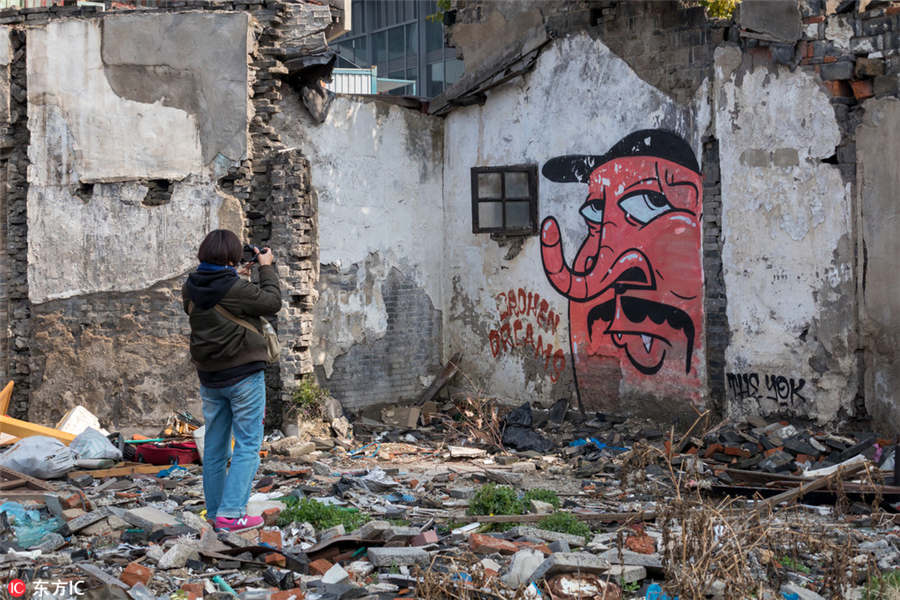In the photograph, a young woman stands on the left side, absorbed in capturing an image of striking wall graffiti with a small rectangular black camera held in both hands in front of her face. She is dressed in pink New Balance shoes featuring a large white "N" on the sides and white soles, blue denim jeans, and layers comprising a black hoodie under a brown jacket. Her short, black hair frames her face as she focuses on the mural in front of her.

The mural, painted on the remaining wall of a severely ruined house, depicts a red-faced man with exaggerated features: a very long, upward-curving nose resembling an elephant trunk, a black cap, and a black mustache. His large eyes gaze to the right, giving a somewhat caricatured, devilish impression. Next to him, partially obscured yet discernible, is the red text "broken dreams."

The setting itself is a desolate scene of ruins and rubble. The house, once white, stands roofless with only one wall remaining intact, while the rest lies in disarray with bricks and debris strewn across the ground. The corner of the house shows a window hinting at its former structure. Below the mural, there's some sort of Asian logo in a red circle with white characters, adding another layer of mystery to this dilapidated environment.